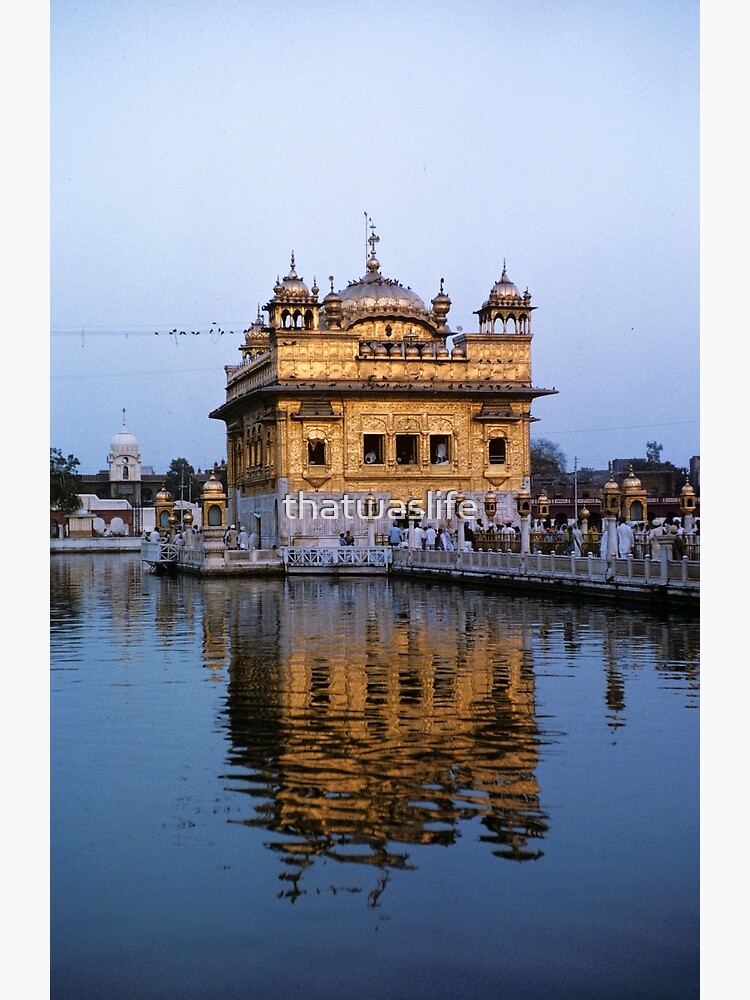A majestic brown castle rises from the end of a pier that juts into a tranquil lake. The castle's lower walls are encased in gray stone, reinforcing its formidable presence. The structure is approximately two to three stories tall, capped by an array of distinctive domes. Dominating the roof is a large central dome crowned with a spike, flanked by two smaller turrets at the corners, each sporting a similar spiked dome.

A short, white post fence runs along the edges of the pier, providing a modest barrier. Surrounding the castle, other buildings with matching round domes and spikes pepper the shoreline, harmonizing with the main structure. The calm waters of the lake mirror the castle's grand features, creating a striking reflection.

Emblazoned on the castle's front wall is the phrase "That Was Life," serving as a haunting inscription. In the background, a verdant forest stretches out beneath a canopy of overcast skies, adding to the scene's mystical and timeless atmosphere.